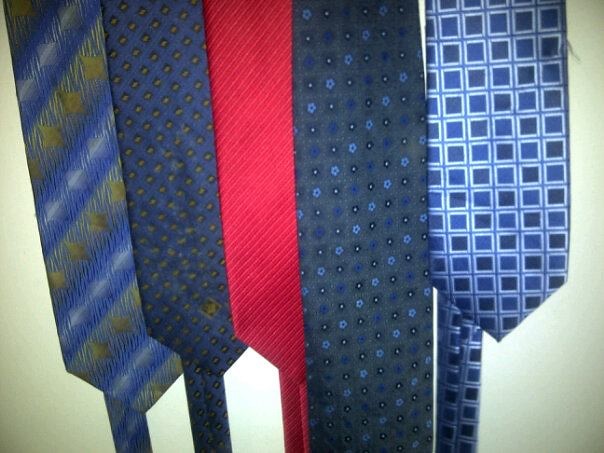The image captures a close-up landscape view of the bottom portions of five men's ties, neatly arranged in a row against a plain, vaguely cream-colored background. These ties, hanging over the edge of an unseen object, dominate the frame with their pointed ends on display. From left to right:

1. The first tie is predominantly blue, featuring diagonal stripes of gold and white, interspersed with star-like and circular shapes.
2. The second tie is a deep navy blue adorned with a pattern of small gold diamonds.
3. At the center is a solid red tie with delicate, raised diagonal lines.
4. The fourth tie showcases a grayish-blue background patterned with a checkerboard of small flowers in varying shades of blue and white centers.
5. The fifth and final tie has a blue and white checkerboard pattern, with dark blue centers and lighter blue outlined squares framed by white borders.

These ties, each with a distinct design, add a vibrant and varied visual appeal to the image.